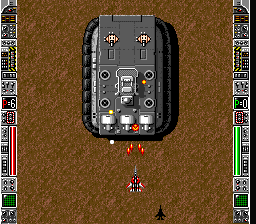The image showcases a retro-style, top-down shooting video game, reminiscent of classic arcade titles from years gone by. The scene depicts a bird's-eye view of a fighter jet engaged in an intense battle against a large, grey gunship, suggesting a potentially climactic boss fight at the end of a game stage. The interface includes various aircraft controls positioned on the left and right sides of the screen, enhancing the authenticity of the shooter experience. The ground below is predominantly brown, evoking the atmosphere of a war-torn battlefield.